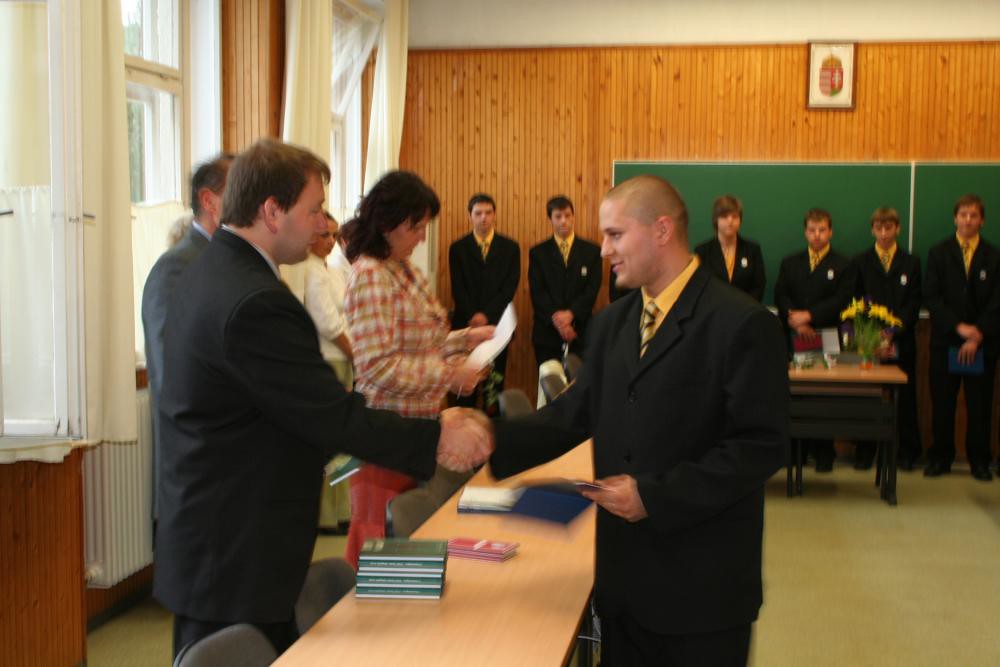In a room with wooden panel walls and a large green chalkboard, a ceremony appears to be in progress. Standing along the back wall are several teenage boys dressed uniformly in black suits, yellow shirts, and yellow and black ties. In front of them is a wooden desk extending from the lower center to the rear center of the room, with a stack of green-covered books and a vase with yellow flowers, possibly daffodils. On either side of the desk, a young person with closely cut hair in a black jacket, yellow shirt, and matching tie shakes hands with an older man also in a black jacket. The young person holds a cell phone in his other hand while they both gaze at each other. Next to the men, a woman with black hair, clad in a white and pink plaid shirt over a red dress, examines a piece of paper. The left side of the room features white-framed windows with white curtains. The scene conveys a formal, solemn atmosphere, suggesting a recognition event or school ceremony.